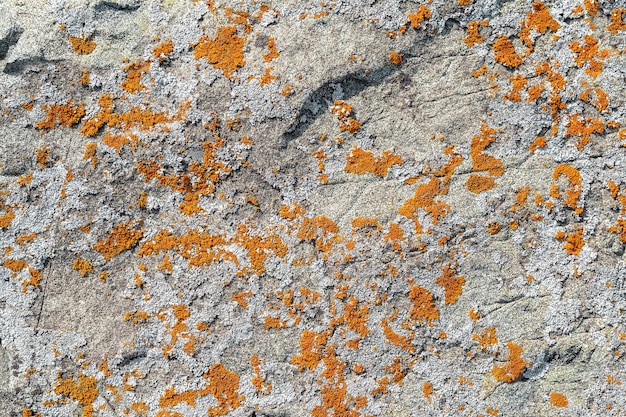The image features a gray rock face that is both smooth and cracked, with noticeable divots and holds, particularly in the upper left and upper center areas. The surface is adorned with vibrant golden yellow and orange splotches that resemble pollen or possibly lichen, scattered across the rock in an irregular, almost Jackson Pollock-like fashion. These speckles vary in size, creating a patchwork effect from top to bottom. The rock face also features a prominent fissure near the center top that resembles the shape of an eye. The overall texture and condition of the rock surface, combined with the colorful splotches, suggest long-term exposure to natural elements, creating a visually dynamic and detailed scene.